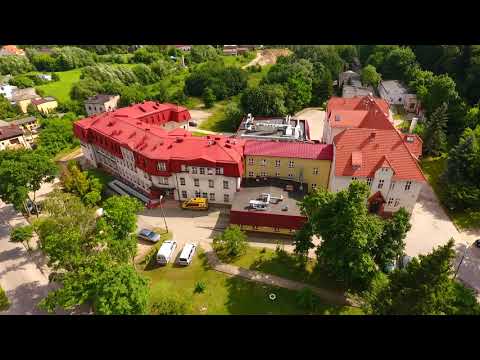This overhead photograph captures a picturesque, tree-nestled resort or hotel complex featuring a prominent series of interconnected, white-walled buildings with characteristic bright red roofs. The central cluster of these buildings forms a U-shape configuration, with the left wing showcasing a relatively flat roofline while the right wing has a distinct peaked roof and a noticeable gable. The main entrance, located within a semi-circular driveway, allows for easy access and drop-off, adding to the welcoming ambiance of the property. Surrounding the central complex is a lush, green landscape dotted with large oak trees and additional smaller buildings made from the same white material but without the red roofs. Towards the bottom left-center of the image, two white vehicles are parked on the vibrant green grass, enhancing the resort's picturesque rural setting. Behind the main buildings lies a grove of trees, which further adds to the serene and inviting atmosphere of the area.